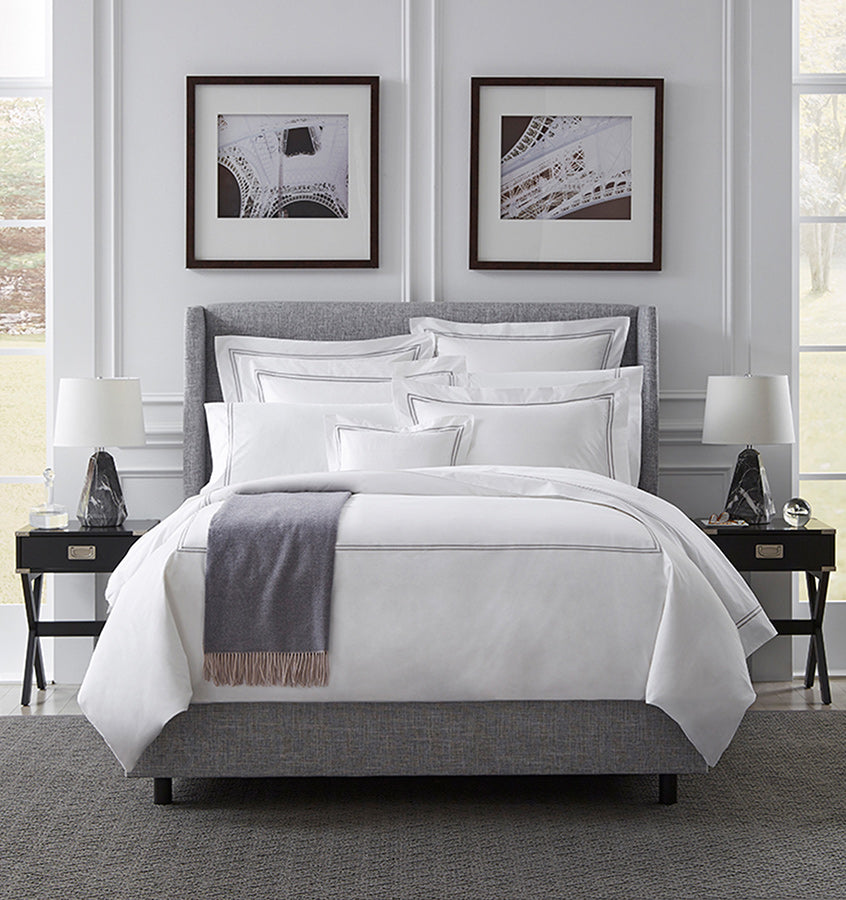This magazine-worthy bedroom features a meticulously made bed with predominantly white sheets adorned with a subtle gray double-lined pattern. The bed is complemented by five pillows bearing the same white and gray double-lined design. Draped over the end of the bed is a dark gray throw blanket with charming tassels. The bed frame is a sophisticated gray, matching the gray carpet underneath. Flanking the bed are two identical black nightstands, each with a silver metal pull handle. On each nightstand rests an identical marble-like lamp with a white lampshade. The right nightstand also holds a glass circle and what seems to be red glasses, while the left features a glass figurine. Above the bed, two black-framed, black-and-white photographs of different perspectives of the Eiffel Tower add a touch of elegance to the white walls. Windows on either side of the bed offer a glimpse into a wooded backyard, further enhancing the serene and luxurious ambiance of the room.